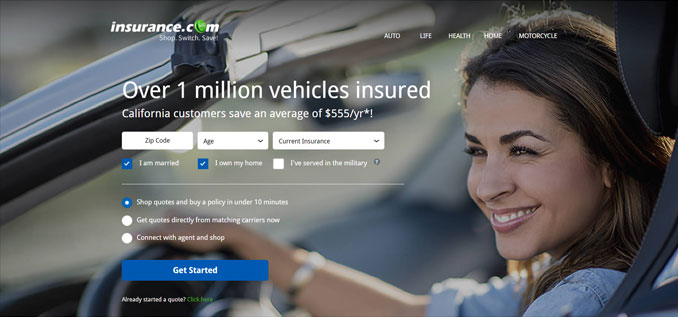In the image, a woman is driving a silver car with the website "insurance.com" displayed prominently at the top of the image. She has a warm smile on her face, thick brown eyebrows, and brown hair. Her right hand rests confidently on the steering wheel, adorned with a silver bracelet, while she glances out the side window. She is wearing a denim top with sleeves rolled up, exuding a casual yet stylish vibe.

The website banner overlaid on the image features the name "insurance.com," with the "O" in insurance highlighted larger and in green. It provides various insurance options, such as auto, life, health, home, and motorcycle insurance. The text also highlights that over 1 million vehicles are insured and that California customers can save an average of $555 per year. Below this, there are white input bars for entering personal information such as zip code, age, and current insurance details.

Additional interactive elements include checkboxes for statements like "I am married," "I own my home," and "I've served in the military," with the first two boxes checked. The banner claims users can "Shop quotes and buy a policy in under 10 minutes." White circles prompt users to "Get quotes directly from matching carriers now," or "Connect with an agent and shop." Finally, a large blue "Get Started" button sits prominently at the bottom, inviting users to begin the insurance shopping process.